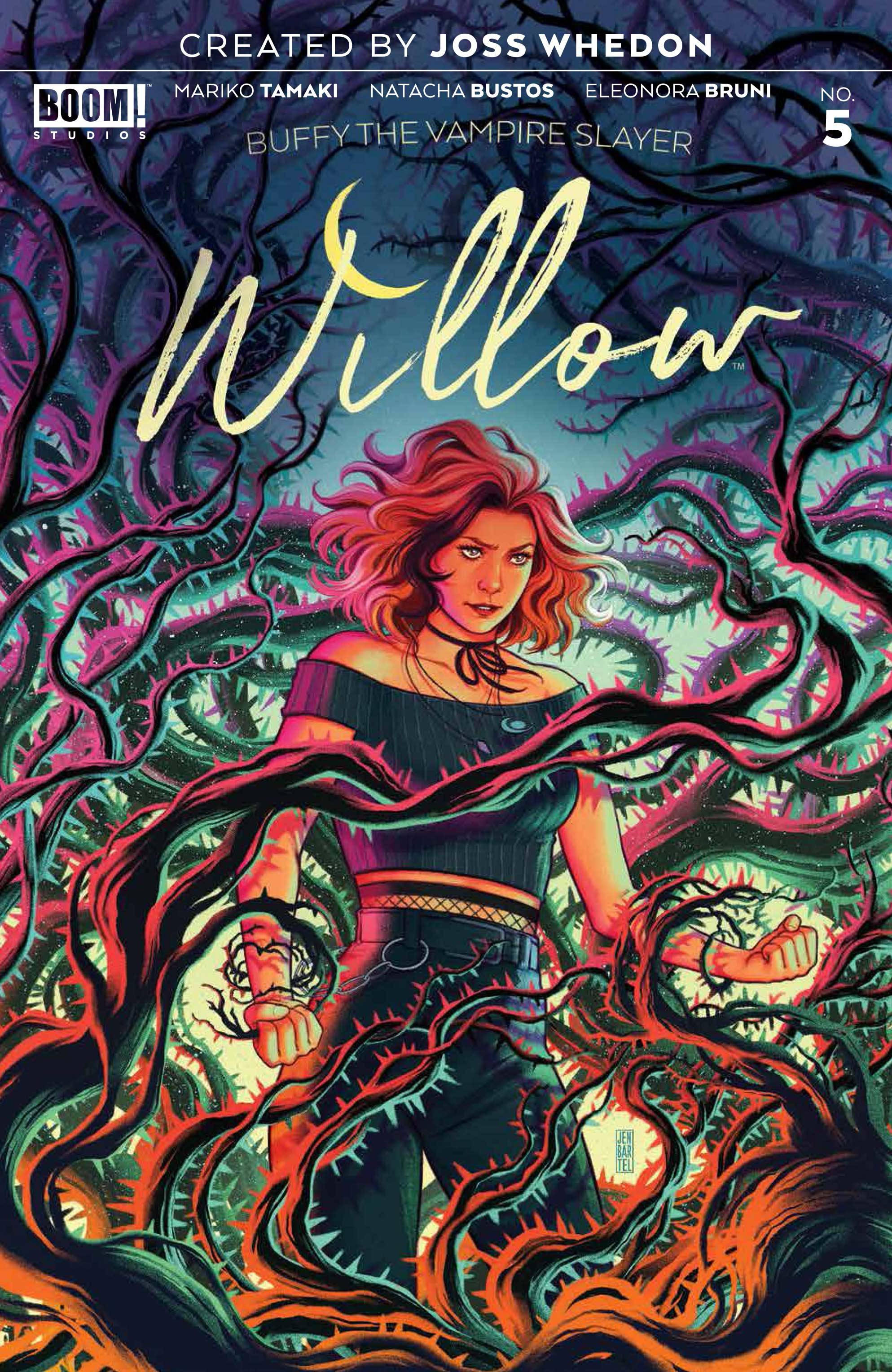The image resembles a comic book cover titled "Willow," featuring a striking, anime-style illustration of a Caucasian girl with light eyes and flowing reddish hair. The character is dressed in an off-shoulder, black crop top, tight black pants, and a belt. She also sports a ribbon around her neck and a necklace. She's surrounded by thorny vines that wrap around her wrists and extend behind her, showcasing shades that transition from orange and light pink to dark purple against a dark blue background that fades to a lighter hue towards the bottom. 

At the top center, in white print, the cover states "Created by Joss Whedon," followed by a thin white line spanning from left to right. Below this line, on the left, is the Boom Studios logo in black on a white rectangle. To the right are the names Mariko Tamaki, Natasha Bustos, and Eleonora Bruni, followed by the number five. Beneath this, in thin yellow print, it reads "Buffy the Vampire Slayer." Dominating the lower section of the cover, in large cursive yellow font, is the title "Willow," with the 'i' dotted by a crescent moon. The overall color scheme transitions from the dark blue at the top to lighter shades as it progresses downward, enhancing the eerie and enchanting atmosphere of the artwork.